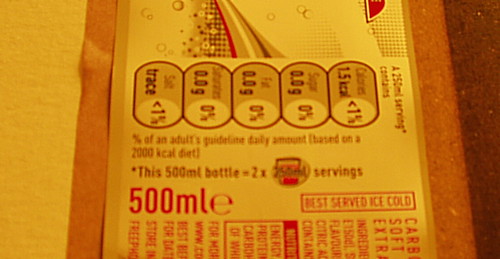The photograph depicts a flat, spread-out product label that appears to have been removed from a beverage container, likely a soda or diet drink. The label, displayed sideways, reveals distinctive features such as a yellow and brown border on the left, progressing to more yellow, red, and brown stripes and stars at the top. Prominent text includes "500 mL" and "best served ice-cold," emphasizing it is for a 500-milliliter bottle, which equates to two 250-milliliter servings. Cues like "1.5 kilocalories" and "trace amount of salt" suggest it is a low-calorie, possibly diet beverage. The logo partially visible is in red, with most lettering, except for nutritional information, presented in black circles. The label rests on a wooden surface, highlighting its flat, removed state.